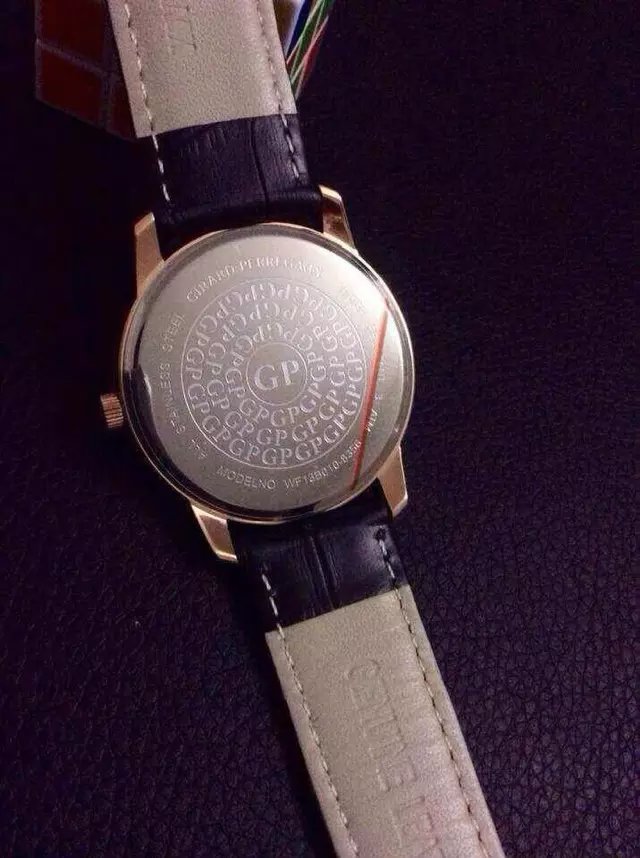The image displays the back of a sophisticated watch, showcasing its intricate design. At the center, there is a prominent circle featuring a bold "G" and "P" side by side. Surrounding these central initials, the letters "GP" are repeatedly arranged in three concentric rows, forming a circular pattern that accentuates the focal point. The watch band starts with a black segment extending about an inch, transitioning to a gray area that encompasses the back of the watch. This gray portion is similarly reflected on the lower part of the watch, separated by small black rectangular sections. The structure appears to be meticulously sewn together at the top and bottom, as well as along the left and right margins. Adding to the complexity, a cluster of wires emerges from the upper section of the watch, adorned in shades of purple, green, and pink, indicating advanced connectivity or internal functionalities.